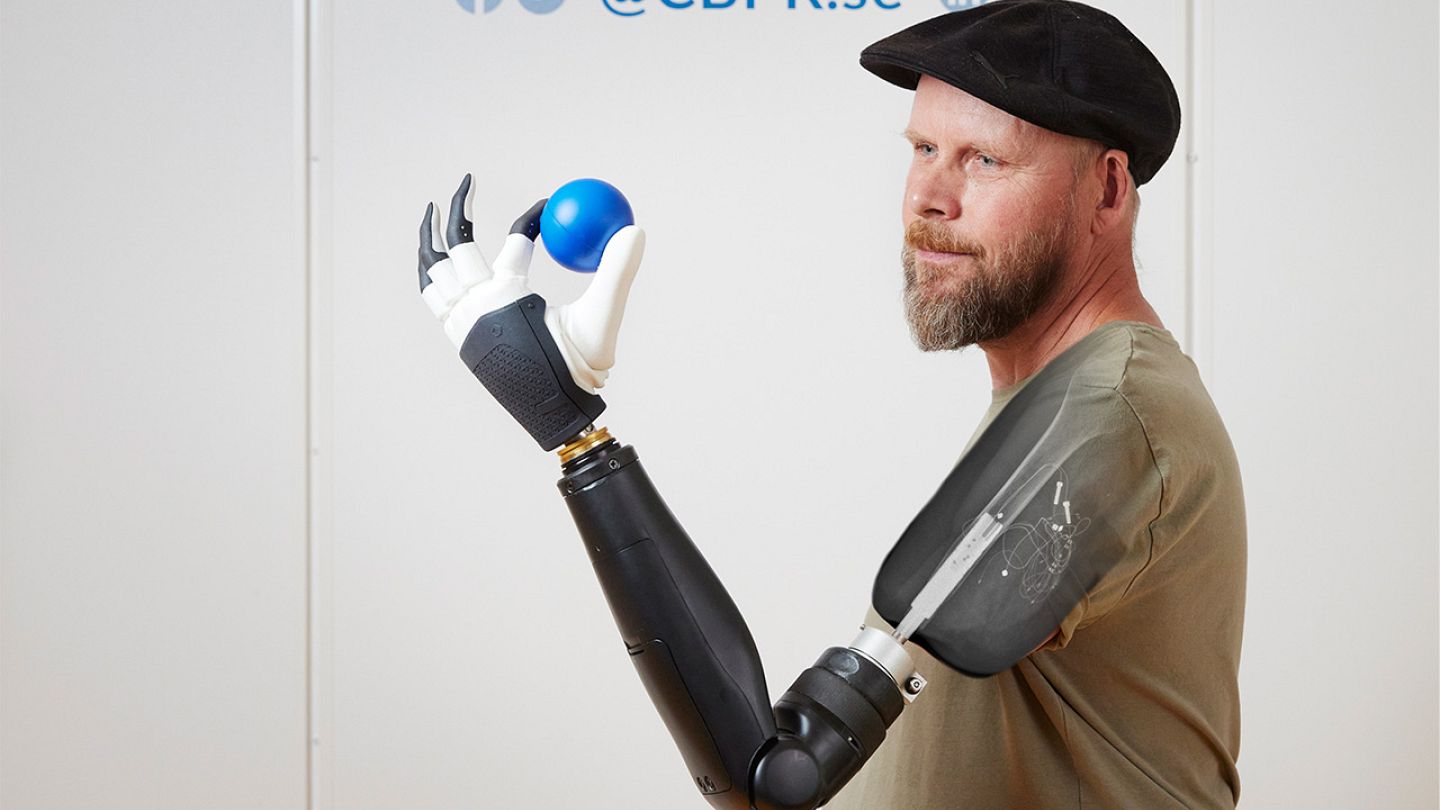This photograph captures a white male amputee, seen in side profile facing left, set against a blank white wall. He dons an olive drab green short-sleeved t-shirt and a black cap, partially covering what might be a bald head. His facial features include a brown beard and mustache. The focal point of the image is his advanced prosthetic left arm, which appears to showcase a blend of black and white components—primarily black with white fingers and black fingertips. The arm is depicted with an x-ray-like superimposition, revealing the internal mechanisms such as wires and connectors that likely interface with his muscles and nerves. Demonstrating the arm’s dexterity, he is precisely holding a small blue ball between the prosthetic index finger and thumb, and he is observing this action with a satisfied expression. The image suggests an advertisement, emphasizing the functionality and life-enhancing capabilities of the prosthetic arm.